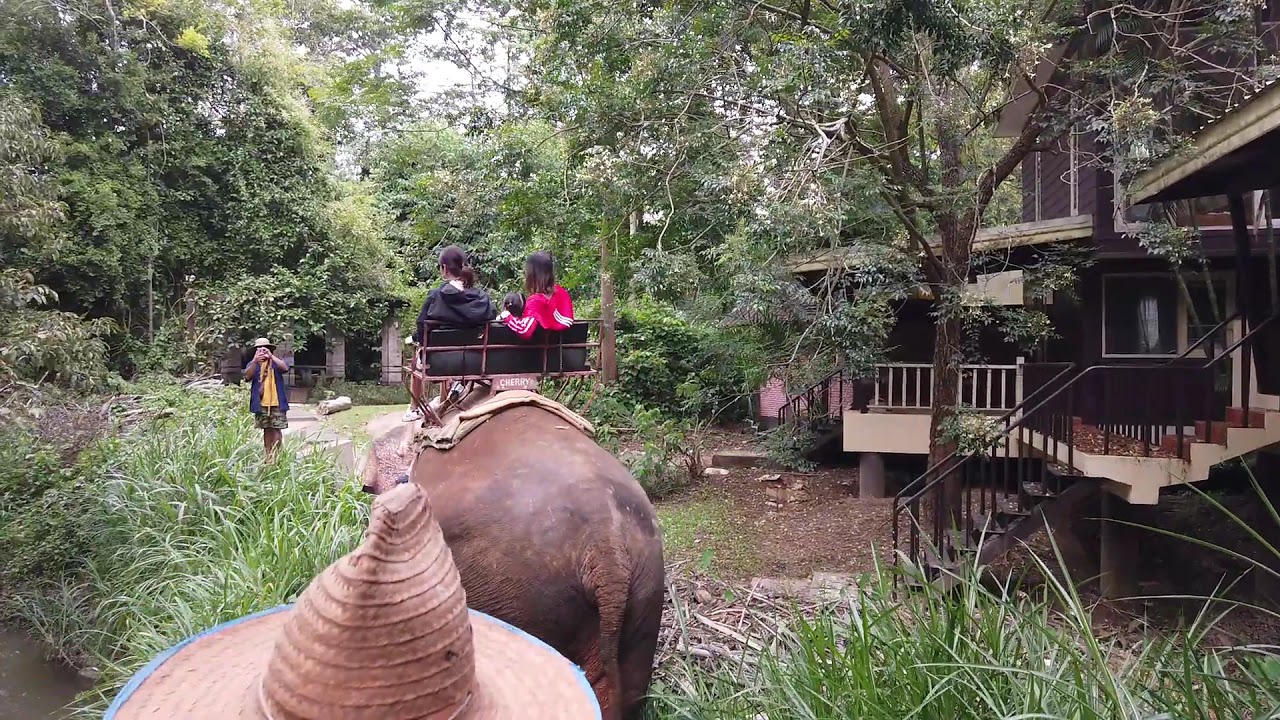The photograph captures a scenic elephant ride, presumably in an Asian tourist destination like Indonesia. The focal point is the rear view of a large, brownish elephant, seen from the vantage point of another elephant directly behind it. On the back of the first elephant, two tourists are seated in a saddle-like chair. The person on the right wears a red hoodie and has long brown hair, while the person on the left sports a black hoodie, with their hair up in a ponytail. Both are accompanied by a child. 

In front of the elephant, a man dressed in a yellow t-shirt, blue vest, red long sleeves, camouflage green shorts, and a white hat is busy taking pictures of the riders. The image also features a portion of a straw hat near the camera, indicating the likely presence of another individual close to the photographer but not fully visible.

The background showcases a modest brown house with stairs, surrounded by lush green trees and high grass, suggesting the area is part of a dense forest. This setting highlights the natural beauty typical of a tourist attraction, immersing visitors in an authentic, outdoor experience.